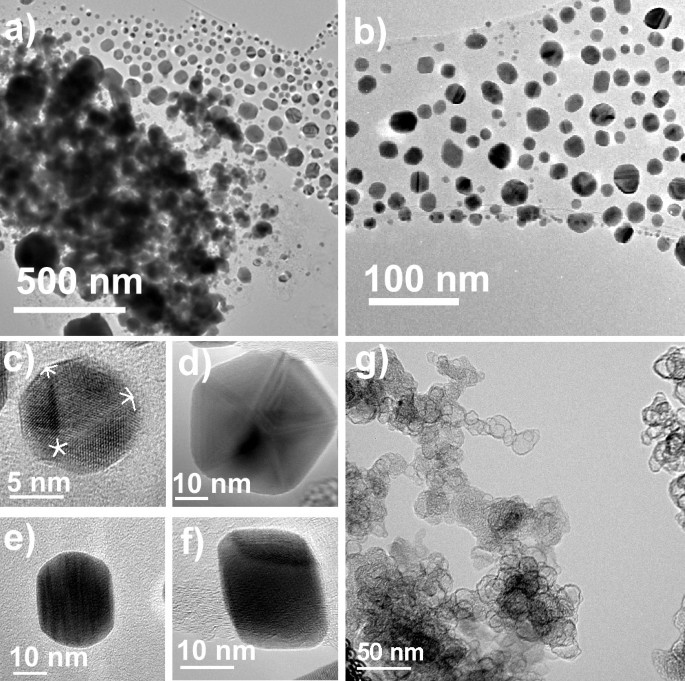The image is a collage of seven black-and-white microscopic photos labeled A through G, showcasing various objects and patterns at nanoscale ranging from 5 nanometers to 500 nanometers. These microscopic photos have been enlarged and each has a scale indicated. Photo A and B on the top row feature hundreds of smaller dots while C, D, E, and F in the middle row display larger, blob-like structures resembling blood drops. G, found on the lower right, shows semi-transparent circles linked together. There's variation in the structures depicted: some clusters of what look like pathogens or bacteria, others similar to fungi, some appearing like pebbles, semi-transparent circles, or even resembling starfish or crystals. The scales provided for each image range between 5 and 100 nanometers, with different composite materials visualized, lending a diverse array of microscopic imagery but without detailed context or labeling for specific objects or organisms.